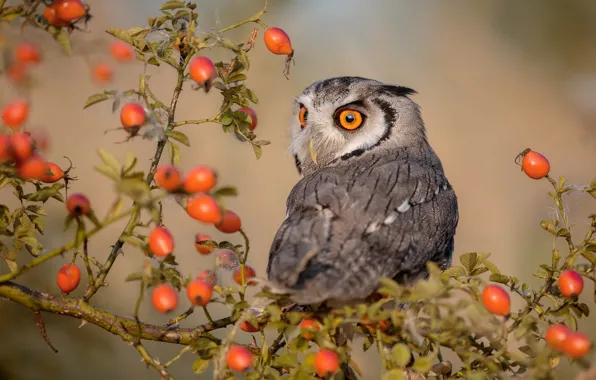This vibrant outdoor color photograph captures a striking scene of a baby owl perched amidst a rose bush laden with clusters of bright orangey-red berries, which have replaced the bush's lost flowers. The background features a soft blur of green, gray, and orange hues. The owl, resting on a small branch, has a captivating appearance with its head turned towards the camera. Its mesmerizing orange eyes with black pupils stand out, complemented by a sharp yellow beak. The owl's head is primarily white and light gray, with subtle black feathering extending outward. Its body displays a pattern of black lines across its back. This detailed and dynamic composition highlights the wildlife in a natural setting, showcasing a rich array of colors including orange, red, gray, black, white, and green, indicating it was taken outdoors during daylight hours.